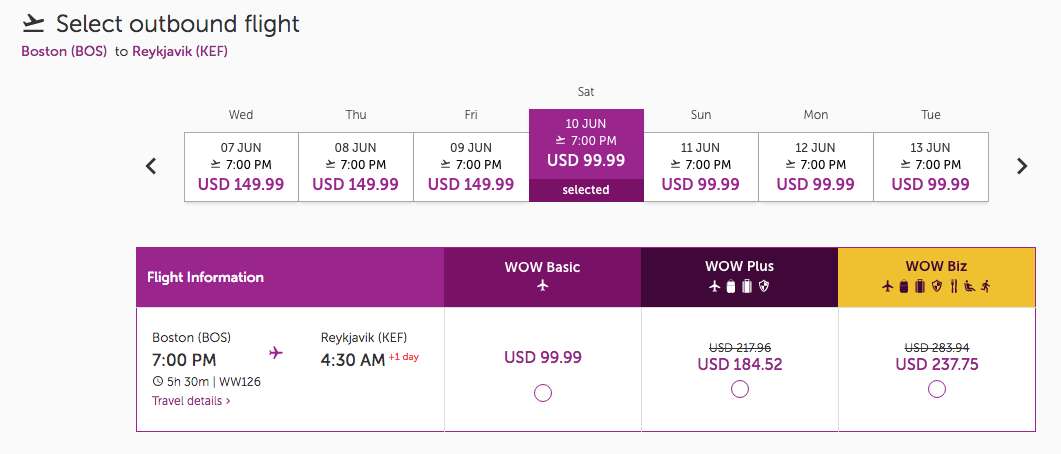The image features a light gray background with text at the top left that reads "Select Outbound Flight" in black. Below that, in purple text, it says "Boston BOS to Reykjavik KEF." Under this header, there are squares labeled with days of the week from Wednesday to Tuesday.

- **Wednesday (07 June)**: 7 p.m. USD $149.99
- **Thursday (08 June)**: 7 p.m. USD $149.99
- **Friday (09 June)**: 7 p.m. USD $149.99
- **Saturday to Tuesday (10 to 13 June)**: All show 7 p.m. USD $99.99

The square for Saturday is highlighted in purple, indicating it has been selected. 

Below the date selection squares, there are four columns labeled "Flight Information," "WOW Basic," "WOW Plus," and "WOW Biz." The first two columns have light and dark purple boxes, respectively; the third column is black, and the fourth column is yellow. The entry in the flight details reads: 
- **Boston 7 p.m.**
- **Reykjavik 4:30 a.m.**